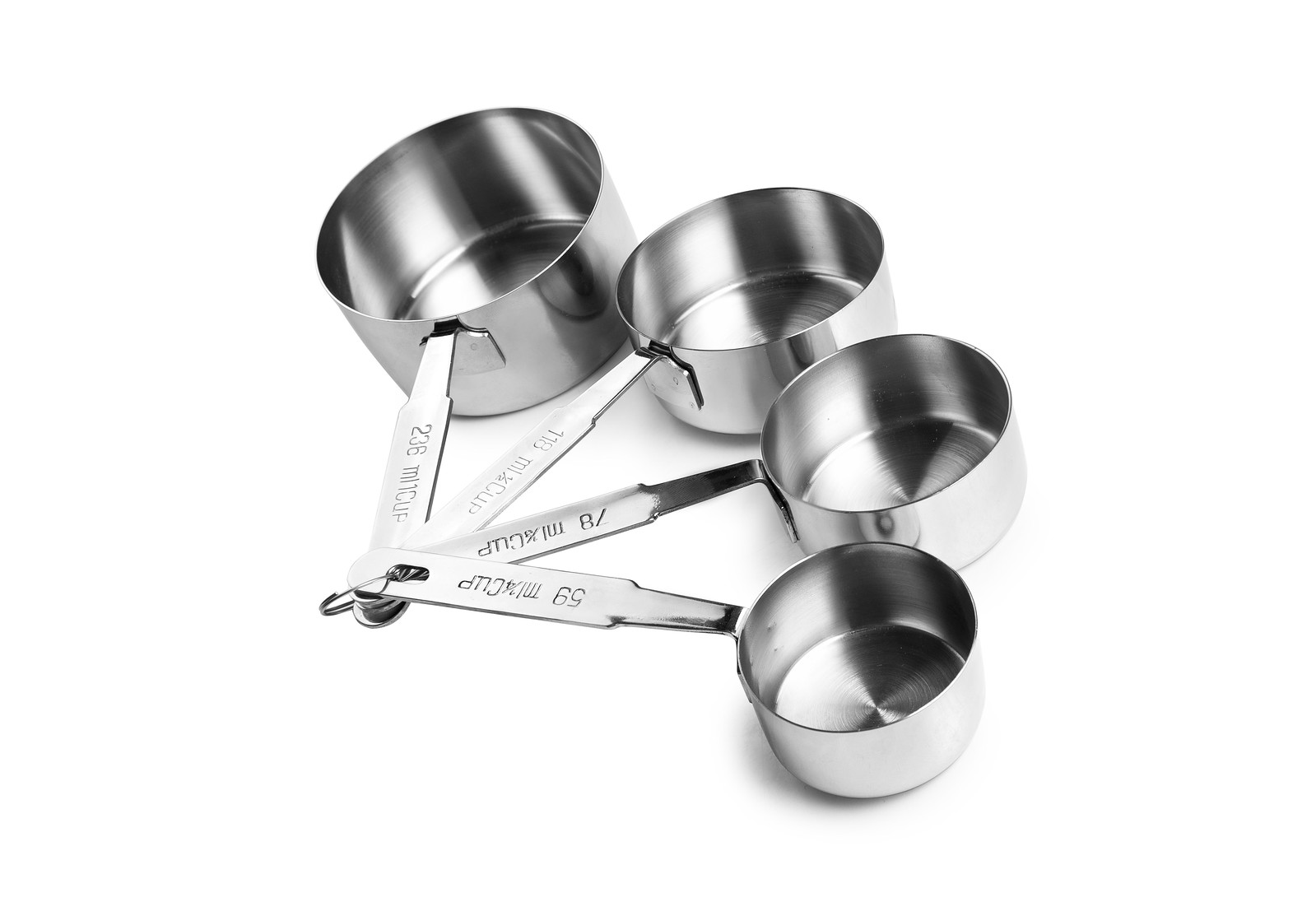The image showcases a set of four stainless steel measuring cups, meticulously arranged against a pristine white background that accentuates their polished metal design. Each cup is connected by a round ring through holes at the end of their handles, allowing for convenient storage. The cups are displayed with their handles oriented towards the bottom left and the measuring parts facing the right, creating a cascading effect from the largest to the smallest. The largest cup is positioned nearly vertical on the left, followed by a cup at one o'clock, then another at three o'clock, and the smallest at four o'clock.

The set includes the following sizes: the largest cup holds 236 milliliters (one American cup), the next size down holds 118 milliliters (half a cup), followed by a 78 milliliter cup (approximately a third of a cup), and the smallest cup holds 59 milliliters (a quarter of a cup). Each cup casts subtle shadows, with a noticeable shadow at the base of the cup positioned at one o'clock. The interior of each cup shows gentle shadowing, adding depth to the image. This clinical and well-lit depiction emphasizes the product's quality and durability, making it ideal for measuring oils, salts, sugars, spices, and other ingredients in cooking.